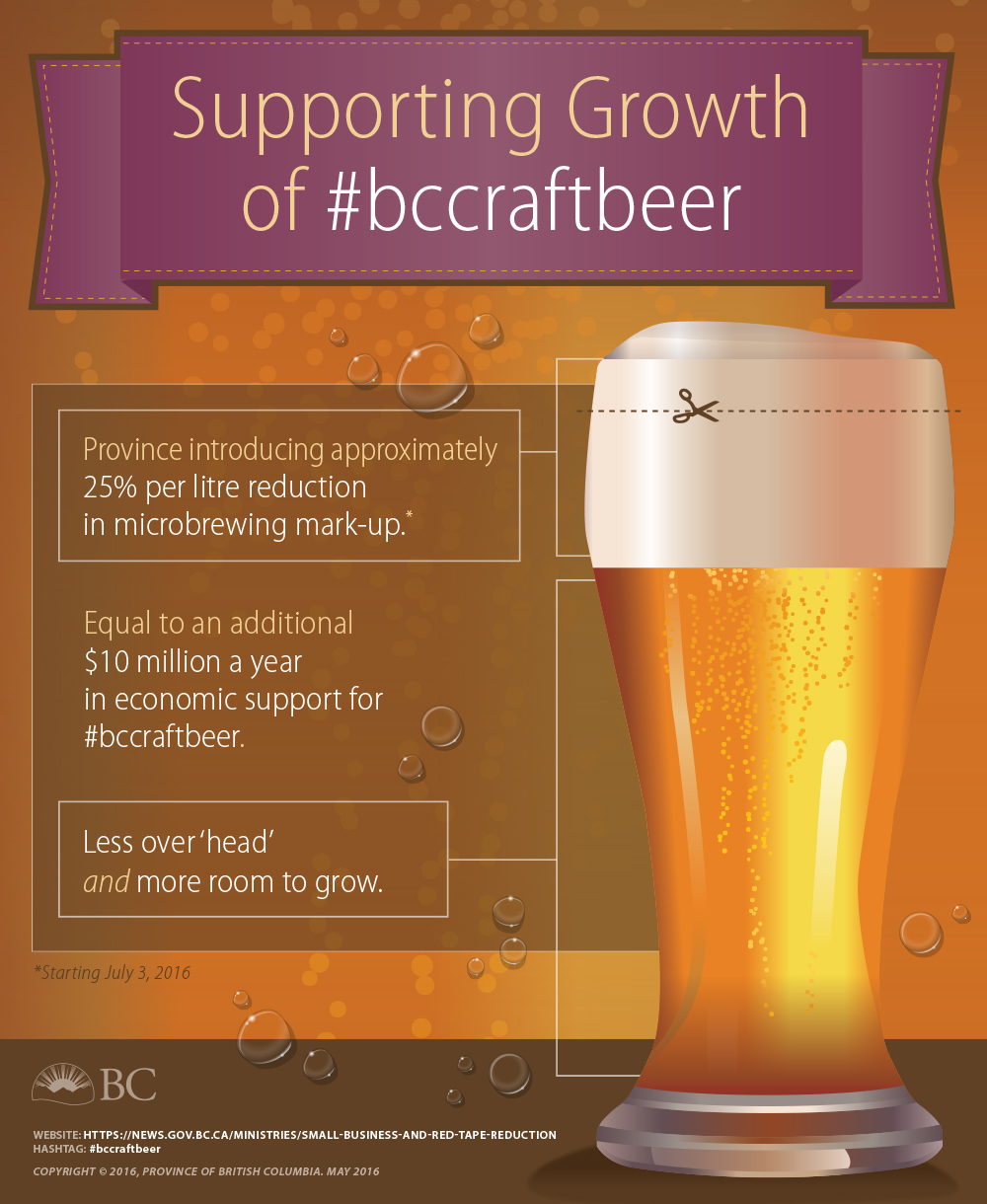This digitally rendered advertisement supports local BC craft beers, featuring a vibrant golden background with bubbles, resembling a glass of beer. At the top, a purple banner with gold and white text reads "Supporting Growth of #BCCraftBeer." Just beneath the banner, on the right side, a foamy tall glass of golden beer is displayed, with droplets on its surface and a dotted line with a scissors icon near the rim. To the left of the glass, a flowchart-like series of text boxes, in gold and white sans-serif font, detail the new economic measures: "Province Introducing Approximately 25% Per Liter Reduction in Micro-Brewing Markup," followed by "Equal to an Additional $10 Million a Year in Economic Support for BC Craft Beer," and "Less Overhead and More Room to Grow." At the bottom left corner, a logo depicting a sun over mountains sits above gray text "BC." This promotional piece highlights British Columbia's support for the local craft beer industry.